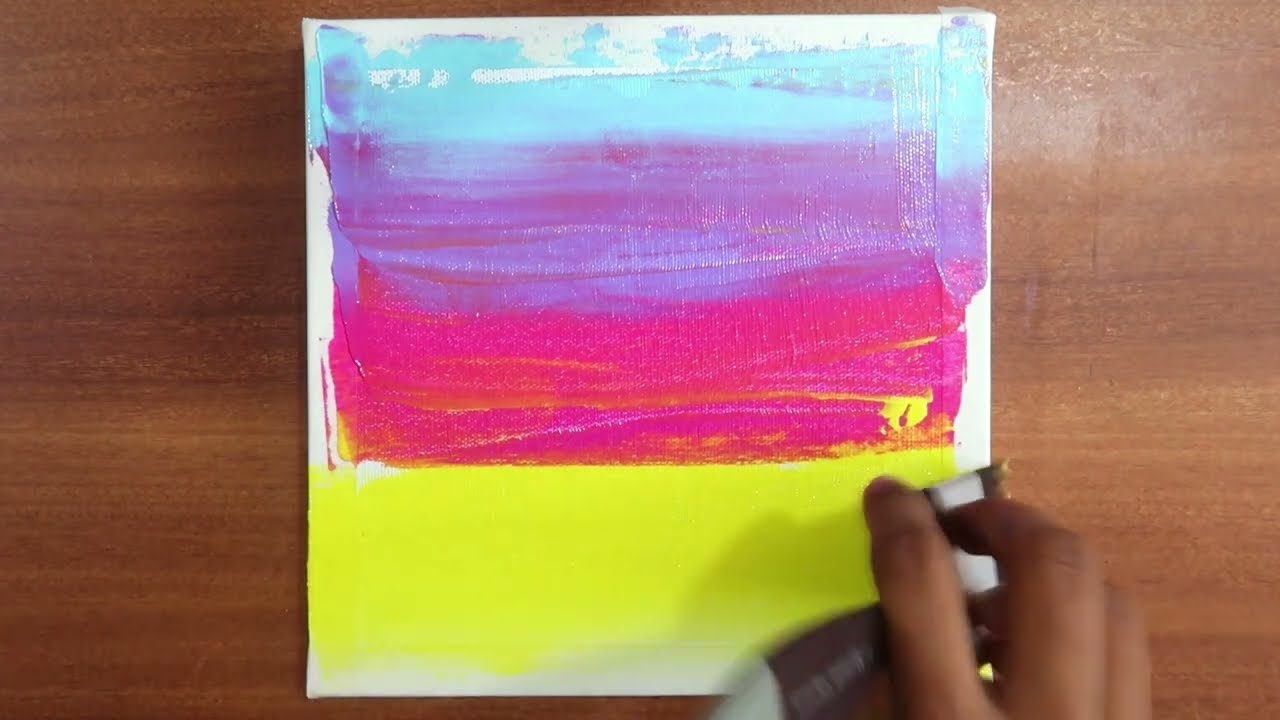In this photograph, a person is painting on a square-shaped white canvas placed at the center of a brown wooden table, which reflects light. The painting features several horizontal strips of vibrant colors: light blue at the top, followed by dark blue, red, yellow, magenta, and purple, with the white of the canvas visible in places. In the bottom right corner, a person's brown hand is visible holding a tool, possibly a marker or paintbrush with a white tip and black body. The hand appears poised to add more colors to the artwork. The setting is simply a focused shot of this creative process, showcasing the serene act of painting.